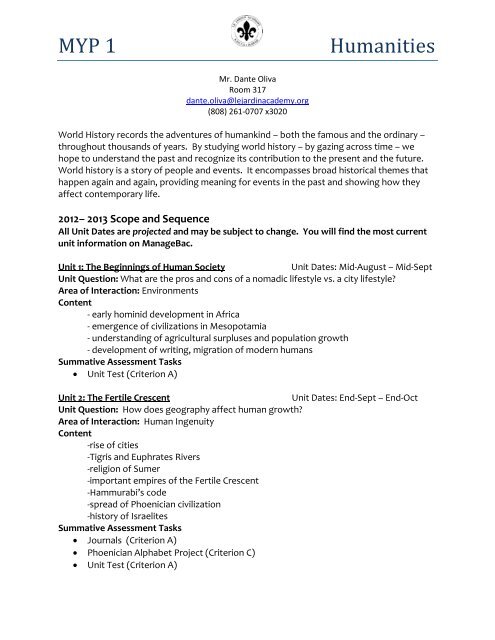The image is a detailed document serving as a syllabus for the MYP1 Humanities class taught by Mr. Dante Olivia in room 317 at Artisan Academy, with contact details including his email (dante.olivia@artisanacademy.org) and phone number (808-261-0707 X 3020). At the top left, the document features "MYP space 1" in blue, followed by a circular emblem. On the right, also in blue, it states "Humanities" with a line underneath. Below this, in black text, the document introduces the course, emphasizing that world history records the adventures of humankind, both famous and ordinary, across thousands of years. It aims to help students understand the past and its contributions to the present and future. The syllabus outlines broad historical themes and their impact on contemporary life. The 2012-2013 scope and sequence section details the units, highlighting that all unit dates are projected and subject to change, with updates available on ManageBac. Unit 1 covers the beginning of human society, addressing topics such as early humanoid development in Africa and the agricultural surplus in Mesopotamia, with assessments including unit tests. Unit 2 discusses the Fertile Crescent, focusing on geography’s impact on human growth and the rise of cities, with assessments including journals and projects on the Phoenician alphabet.